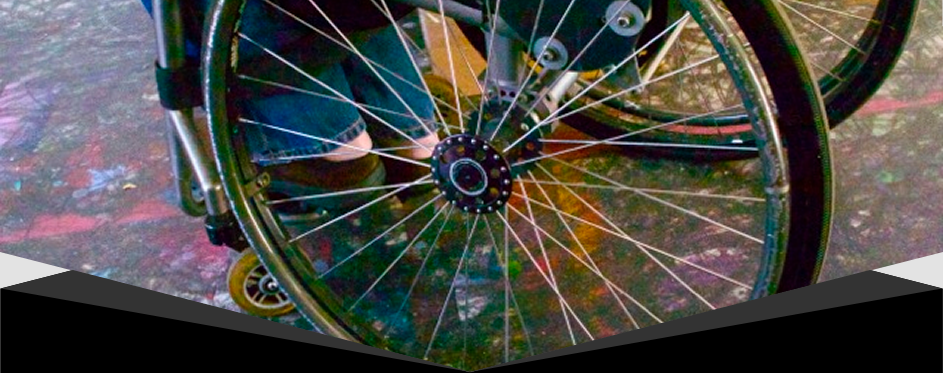The detailed photograph captures the bottom portion of a manual wheelchair on a vibrant, colorful pavement that resembles a mosaic or paint splatter. The pavement exhibits a sunburst prism effect with a spectrum of colors including red, purple, green, yellow, and orange. The image prominently features the left wheel of the wheelchair in the foreground and the right wheel in the background, both equipped with spokes. The legs and feet of the wheelchair user are visible, showing brown shoes with black soles and jeans but no socks. A little bit of the person's ankle is evident as they rest their feet on the wheelchair's leg supports. Additionally, the lower part of the image features a black, wedge-shaped wall pointing toward the center, framing the vibrant scene. This detailed composition captures both the functionality of the wheelchair and the striking, artistic backdrop of the pavement.